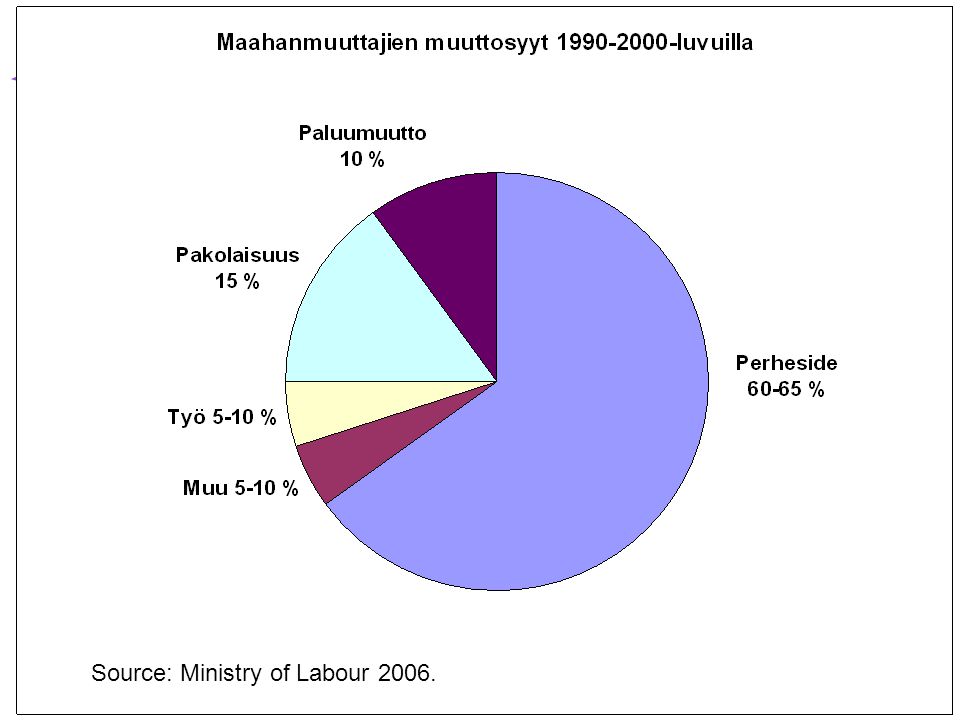The image depicts a pie chart labeled in a non-English language, titled "Mahan Muta Tijian Mutasit 1990-2000 La Vuela," with data sourced from the Ministry of Labor in 2006. The chart is divided into five distinct color-coded segments against a white background with black text. The largest portion, comprising 60-65% of the chart, is shaded in a light lavender color and labeled "Parasite." The second-largest segment, representing 15%, is a bright turquoise color labeled "Pacillus Pacillus." A dark violet section, which accounts for 10%, is marked "Palamuto." Two equally sized segments, each taking up 5-10% of the chart, are labeled "Tayo" and "Mu," colored light yellow and maroon, respectively. The overall arrangement and percentages provide a detailed visual representation of the data from the specified time period.